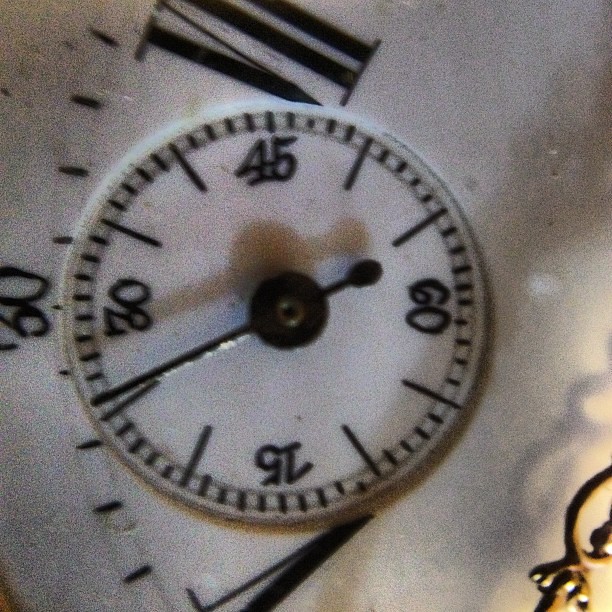This image showcases a very close-up, slightly fuzzy macro photograph of a timepiece, likely a pocket watch or grandfather clock face. The main clock face features Roman numerals, with the numbers V (5), VI (6), and VII (7) clearly visible. There's a distinctive small seconds dial, present within the larger clock face, which is marked at one-second increments with longer marks at five-second intervals and labeled at 15, 30, 45, and 60 seconds. The small black second hand is positioned around the 25 to 26-second mark. Amidst these details, a brass clock hand can be seen in the lower right corner of the image. The entire setup is analog, with a particular emphasis on the intricate detailing of the second markers and the unique overlay of the main and secondary dials.